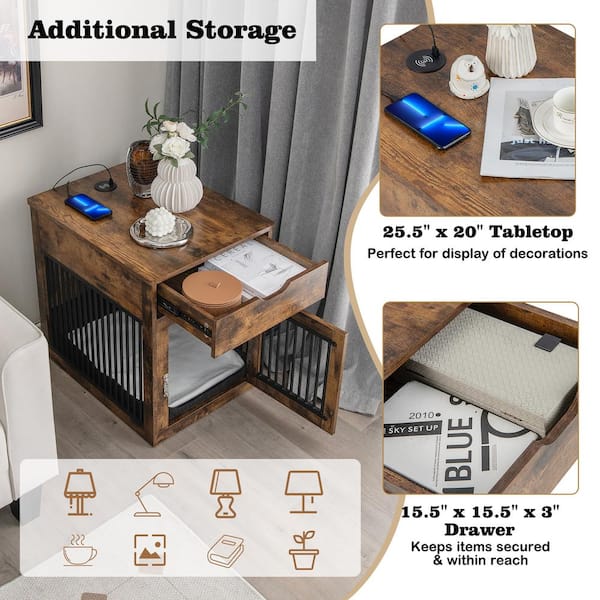This advertisement showcases a dual-purpose pet crate and end table made from medium brown wood. The multifunctional furniture is illustrated through three images. The first image displays the pet crate with an open door revealing a cozy blanket inside. The top functions as a 25.5 by 20-inch tabletop, ideal for displaying items like lamps, books, plants, and coffee mugs. The second image highlights the additional storage feature with a 15.5 by 15.5 by 3-inch drawer that contains a notepad and a container, emphasizing its capacity to keep items secure and within reach. The third image reiterates these functionalities with visual icons and text boxes noting the various decoration options and measurements. Overall, this pet crate end table is perfect for both pet containment and stylish home storage.